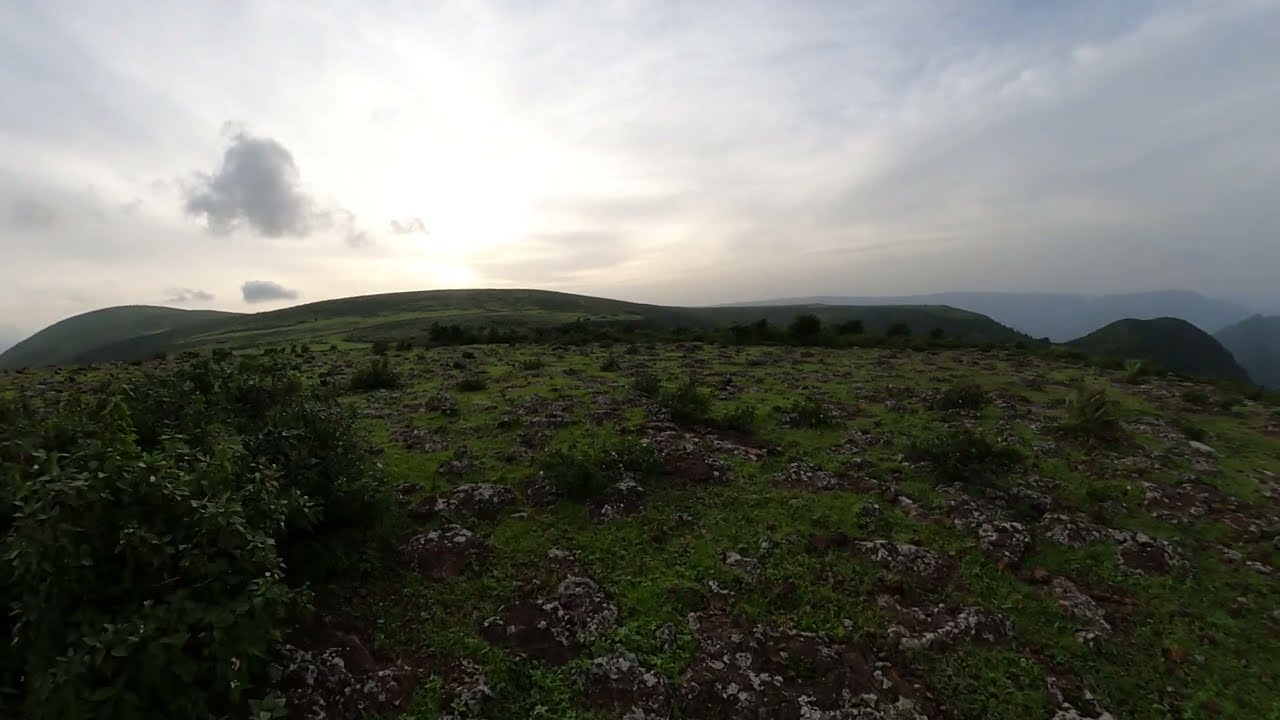A photograph captures a tranquil, hilly landscape as dawn breaks. The image is predominantly dark, owing to the early morning lack of sunlight, which casts the foreground in shadow. The rolling hills are covered in short green grass and scattered with patches of white and brown rock, interspersed with leafy green bushes and shrubs. A brilliant, whitish-yellow sunrise peeks over a hill just left of center, radiating light that contrasts starkly with the otherwise steel-blue and gray sky filled with varying cloud formations. Distant valleys rise into additional hills on the far horizon, lightly shrouded in mist, enhancing the serene and untouched nature of the scene. The landscape is devoid of human presence, making it a purely natural and tranquil sight.